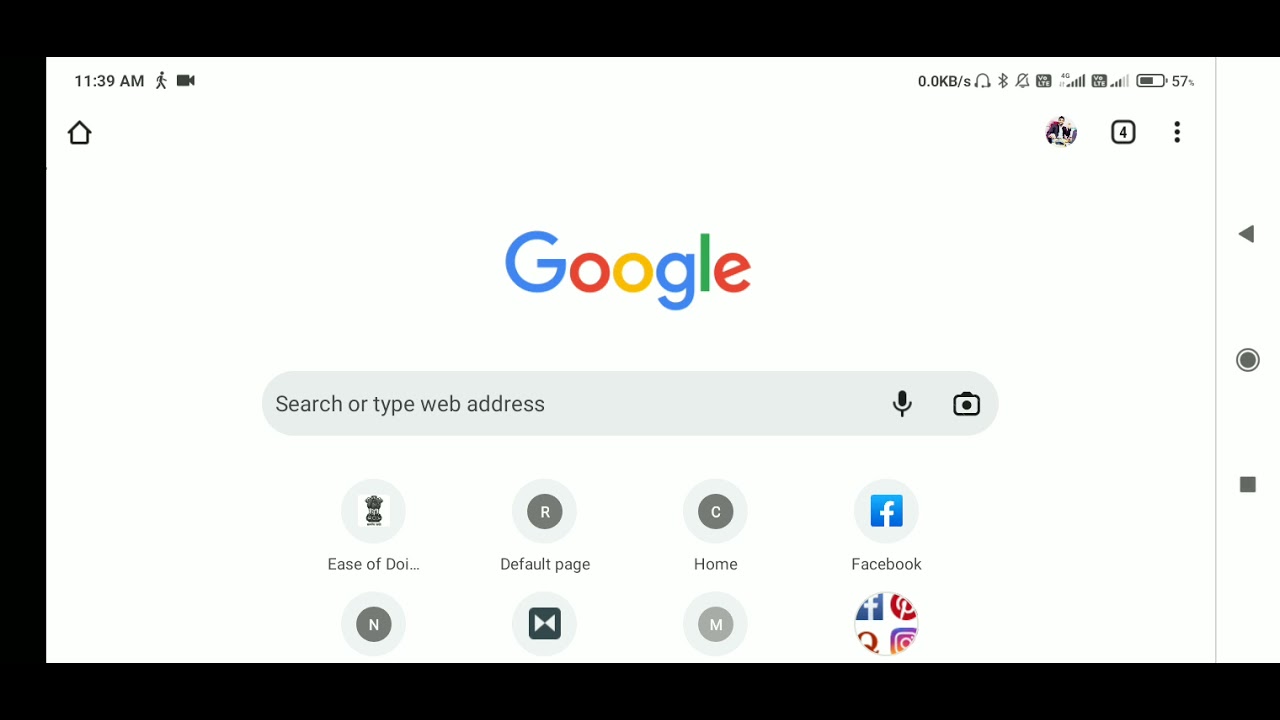The photographic image is a screenshot of a mobile device captured at 11:39 a.m. The status bar at the top displays full carrier signal bars, an active Wi-Fi connection, an alarm bell icon, and a battery life of 57%. Below the device's status bar is a white-background web page interface. 

In the upper left corner of the web page, there's a black home icon. Adjacent to it on the right is a circular profile button featuring an image of a gentleman. Continuing to the right, there's a square button displaying the number "4" accompanied by three vertical dots. 

Centered below these icons is the Google logo rendered in its standard blue, red, yellow, and green colors. Beneath the logo is a search bar with greyed-out placeholder text that reads, "Search or type web address." To the right of the search bar are a microphone icon and a camera icon for voice and image search functionalities.

Lower on the page, a series of eight circular icons display recently searched items. Among them, a blue Facebook icon is prominent. The others include circle icons for Pinterest, Quora, and Instagram, each using their respective platform colors and symbols.